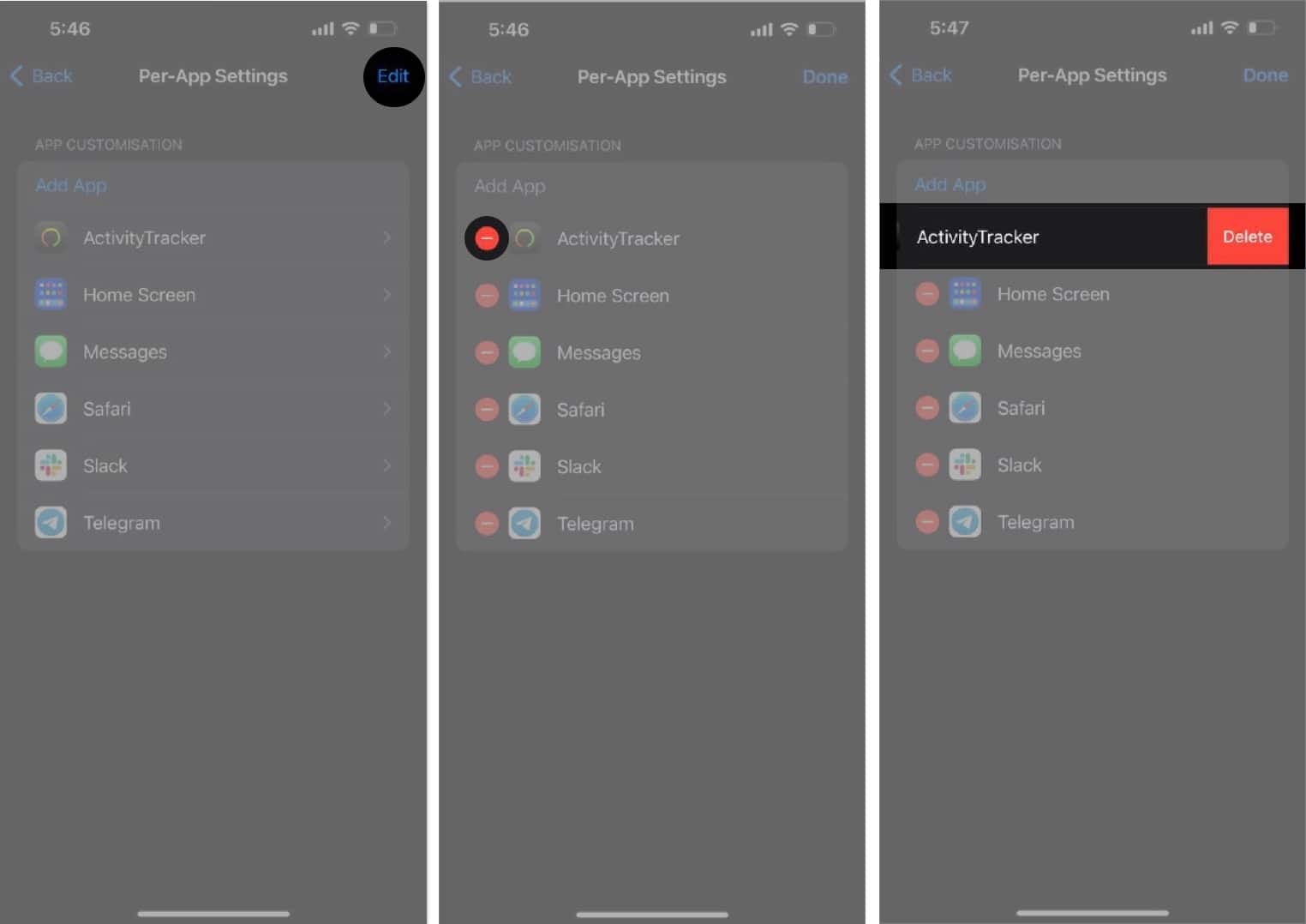The image portrays a collage of three sequential phone screenshots, each taken at either 5:46 PM or 5:47 PM, showcasing consistent Wi-Fi, data strength, and battery levels across all images.

**First Screenshot (5:46 PM):**
This screenshot highlights the home screen with various apps displayed, including "Activity Tracker," "Home Screen," "Messages," "Safari," "Slack," and "Telegram." At the top, you can see icons for the back button and "per app settings," as well as an "App Customization" option. The interface appears to be set for app management functions.

**Second Screenshot (5:46 PM):**
The same list of apps appears here, but with a red delete icon next to each, suggesting the user has entered the app deletion mode. Notably, a black circle is drawn around one particular app, demonstrating the selection process for deletion.

**Third Screenshot (5:47 PM):**
In this screenshot, the "Activity Tracker" app is specifically highlighted. A red "Delete" button appears on the right side, indicating that the selected app is ready to be deleted if the user confirms the action. This step-by-step visual guide effectively illustrates the method for deleting an app from the phone.

This triptych offers a clear tutorial on how to delete apps from a smartphone, with each screenshot meticulously demonstrating the sequential steps involved.